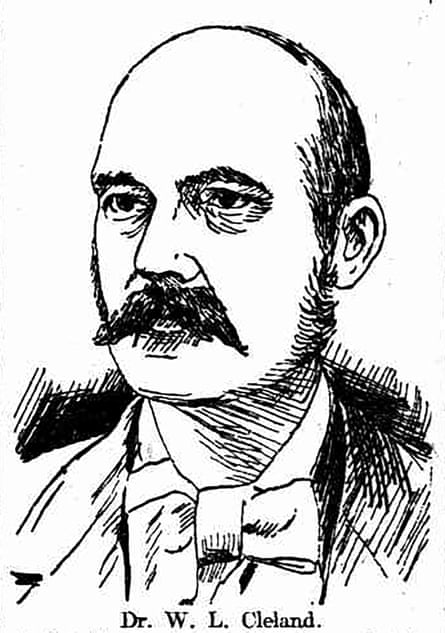The image is an upright, vertical rectangle sketch of Dr. W. L. Cleland, depicted from the chest up. The crisp black lines on a white background suggest it is a simple yet detailed pencil or ink drawing, reminiscent of an 1800s style illustration. Dr. Cleland, a balding man with prominent sideburns and a thick mustache, gazes towards his right. He is dressed formally in a suit with a bow tie. The text "Dr. W. L. Cleland" is inscribed at the bottom of the portrait. The intentional contrast in shading, with his suit being more white on the left and more black on the right, adds depth to the image. The background is fuzzily sketched, leaving it somewhat ambiguous.